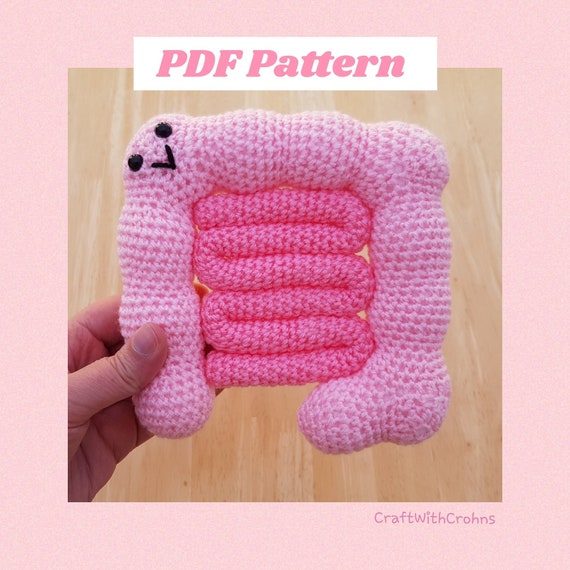The image features a detailed crochet pattern with a whimsical design of intestines, aimed at blending craft and humor. At the top of the image, “PDF Pattern” is prominently displayed in pink letters against a white rectangle. The central focus of the picture is a yellow square showcasing the crochet pattern of intestines, held by a pale-skinned hand, likely of a Caucasian individual. The intestines, crafted in bright pink yarn, feature a lighter pink border and are adorned with a charming smiley face with black eyes and a smile. The playful design appears humorous and might be intended for raising awareness or showing support for individuals with Crohn's disease. The text "Craft with Crohn's" is located at the bottom right corner in pink letters against the solid pink background, suggesting the potential link to Crohn’s disease, either for fundraising or as a thoughtful, supportive gift. The background beneath the crochet pattern is a light tan, hardwood laminate floor, further emphasizing the intricate and colorful yarn creation.